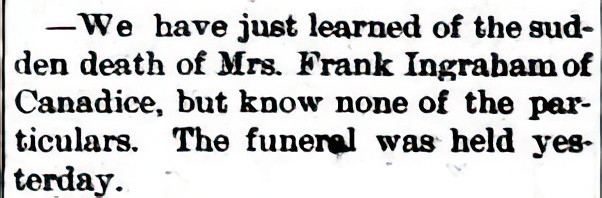The image features a white background with black text that appears to be typed in a typewriter-style font, resembling Times New Roman. The text starts with a dash and reads: "We have just learned of the sudden death of Mrs. Frank Ingraham of Canadese, but none of the particulars. The funeral was held yesterday." The text is slightly grainy and smudged in places, giving it an old-fashioned appearance, and is bordered by thin black vertical lines on both sides. The overall look suggests it could be a photograph of a vintage newspaper clipping or note.